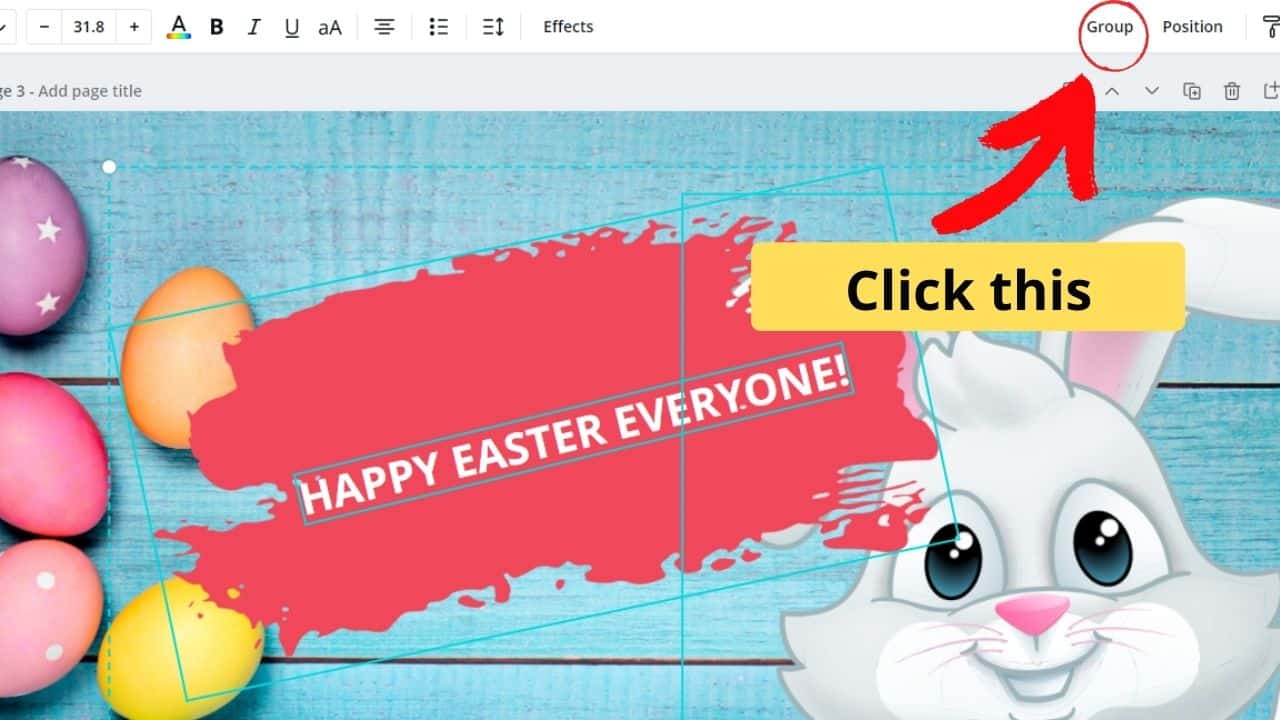The image is a colorful, cartoonish Easter greeting. Dominating the center is a cheerful, big-eyed Easter bunny with a pink triangle nose and a slightly open, smiling mouth. The gray bunny is set against a vibrant red background, with large white text displaying the message "Happy Easter, everyone."

To the right, there's an upward-pointing arrow directing attention to the circled word "group," with the word "position" situated beside it. To the left, the number "31.8" is flanked by a minus and plus sign. Underneath, there is a series of text formatting symbols: a multicolored line beneath the letter "A," a bold letter "B," the letter "I," an underlined letter "U," a lowercase "a" next to an uppercase "A," and a set of five stacked horizontal lines. Additionally, three horizontal lines are followed by an arrow, leading to the word "effects."

To the left of the bunny is an array of brightly colored Easter eggs. The eggs are decorated in various patterns: one is purple with white stars, another is orange, a third is pink, followed by a light pink egg adorned with white dots, and lastly, a yellow egg. The overall tone of the image is playful and festive, capturing the joy of the Easter holiday.